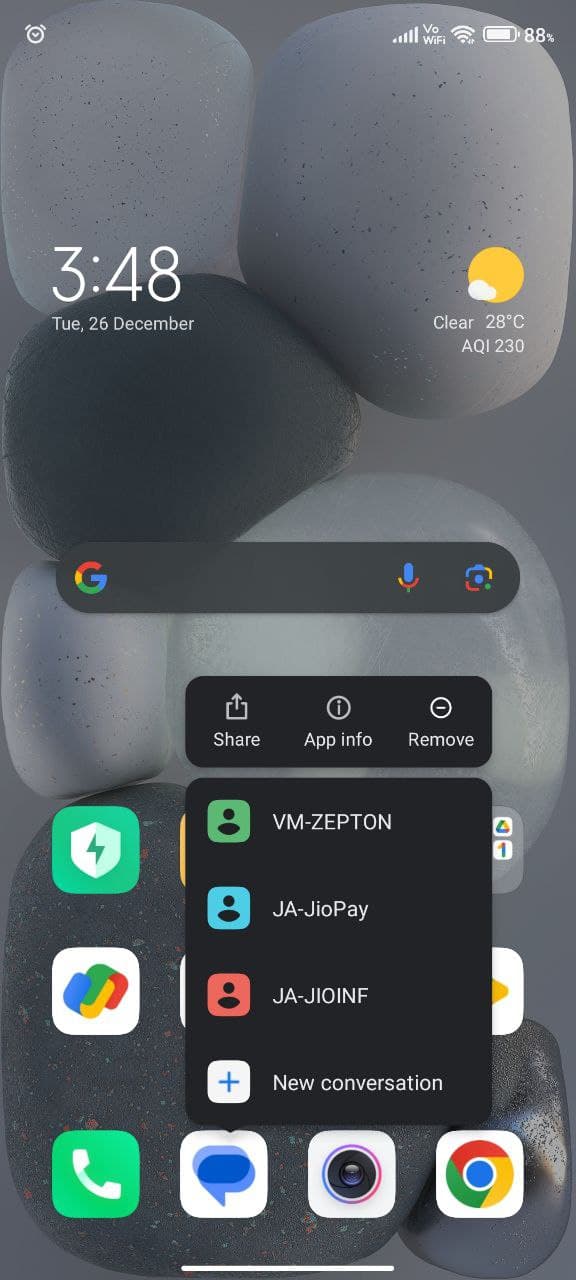A screenshot of an Android mobile phone's home screen, captured at 3:48 AM, with the battery level at 88%. The weather is displayed as a clear day with a temperature of 28°C, indicating a European location. The home screen showcases several app icons including the telephone, messaging, camera, Google, antivirus, and Google Drive apps. The user has long-pressed on an app, revealing a dropdown menu with options to 'Share', 'App info', and 'Remove'. Additionally, the screenshot shows various Bluetooth connections or statuses labeled as "VM-Zeptyn", "JA-GIOP", and "JA-GIOINF", alongside a prompt for a 'new conversation', possibly related to chat messages.